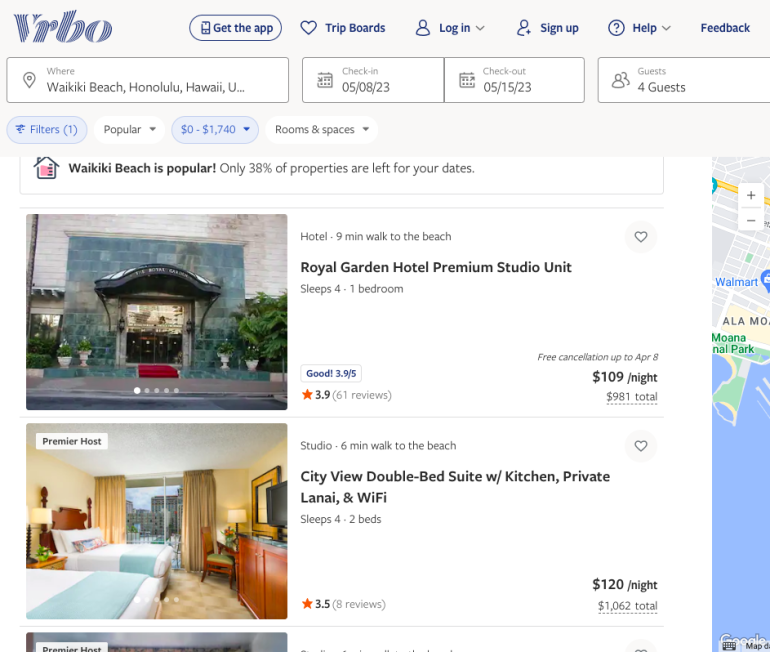In this image, a smartphone screen displays the VRBO app with a clean, primarily white or off-white background. At the very top, an off-white banner stretches across the screen from left to right. The banner features the VRBO logo in a blue font on the top-left corner, followed by several navigation options: "Get the App," a heart icon labeled "Trip Boards," a person icon for "Log In," another person icon for "Sign Up," a circle with a question mark for "Help," a dropdown arrow, and "Feedback."

Below the banner, a white search box reads "Waikiki Beach, Honolulu, Hawaii" as the selected destination. The check-in date is set for May 8, 2023, and the check-out date for May 15, 2023, with a total of four guests. Beneath this search box, various filters are available for refining the search.

A message indicates the popularity of Waikiki Beach, noting that only 38% of properties are left for the selected dates. The first search result listed is for "Royal Garden Hotel Premium Studio Unit," accompanied by an image of the hotel on the left side of the screen. The rate is displayed as $109 per night. Further down, another entry shows an image next to the description "City View Double Bed Suite with Kitchen, Private Lanai, and Wi-Fi," offering additional accommodation options.